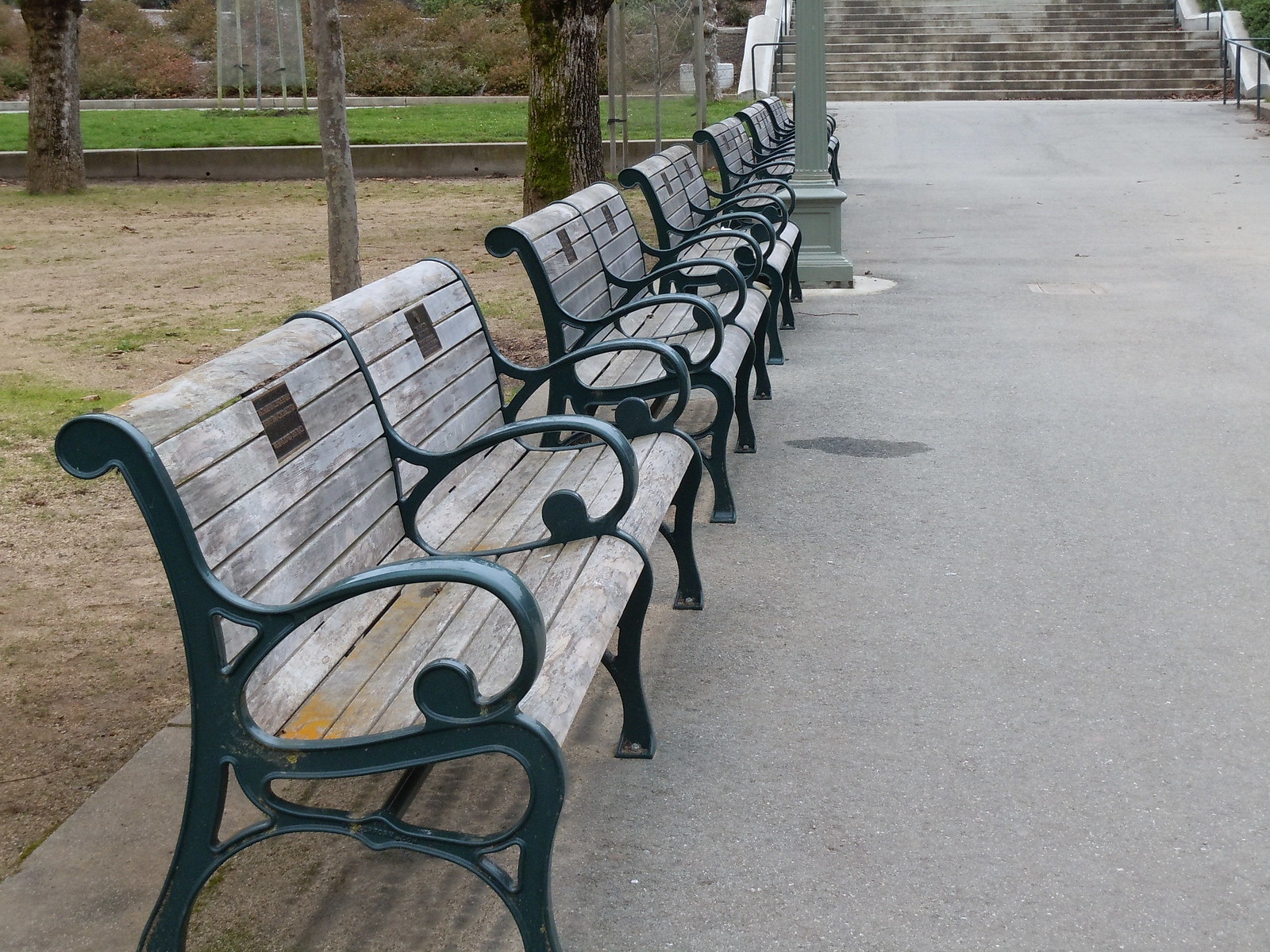This photograph captures a row of six benches situated in a park-like setting. Each bench is designed to seat two people, divided by a central armrest, making three arms per bench—two on the sides and one in the middle. The benches have a sturdy metal frame, likely cast iron, painted either black or green, with gently curved wooden slats for the seats and backs, exhibiting a weathered brownish-gray hue. These benches, with individual plaques on the upper backrest of each seat, are aligned closely together, stretching into the distance.

In the foreground, grey asphalt is visible on the right side, while patches of brown and green grass flank the benches on the left. Tree trunks stand behind the benches, adding to the serene park atmosphere. At the upper part of the image, wide steps lead up to a building, hinting at a frequented public space. The scene evokes a peaceful, inviting environment perfect for rest or contemplation.